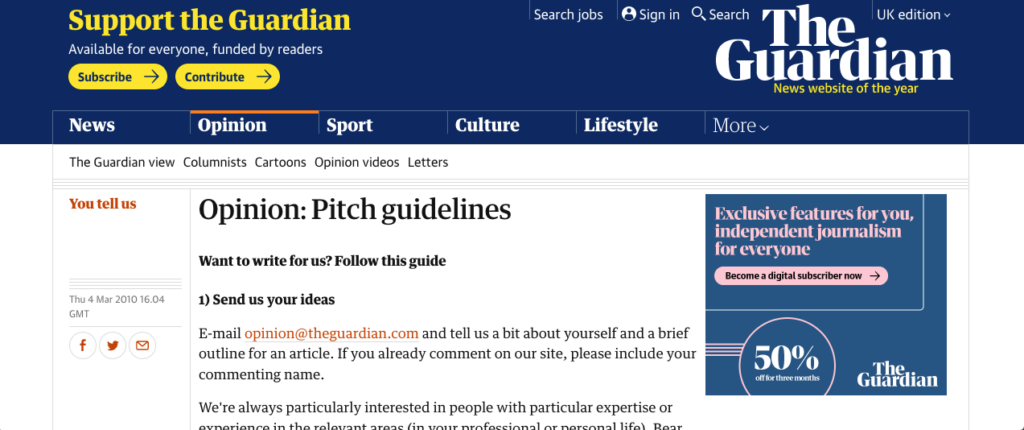This image displays the homepage of The Guardian, an online news website, with its prominent branding at the top. The top banner features "The Guardian" in large white text, accompanied by the tagline "News website of the year" in smaller yellow text. The UK edition is currently selected, but users can switch editions via a dropdown menu. Options to sign in, search, and search for jobs are also available at the top.

On the top left, a prominent yellow banner encourages readers to "Support The Guardian," with the message "Available for everybody, funded by readers." Below this, there are two yellow buttons labeled "Subscribe" and "Contribute."

The main navigation bar includes sections for News, Opinion, Sport, Culture, Lifestyle, and more. The Opinion section is active, indicated by an orange line above it. This section provides pitch guidelines for aspiring writers, advising them to send ideas via email, include a brief description of themselves, and mention any previous comments made on the site.

On the left side, there's a highlighted prompt titled "You Tell Us" from March 4th, 2010, with sharing options via Facebook, Twitter, and email. To the right, an advertisement offers a half-off subscription deal for digital access to The Guardian, promoting independent journalism.